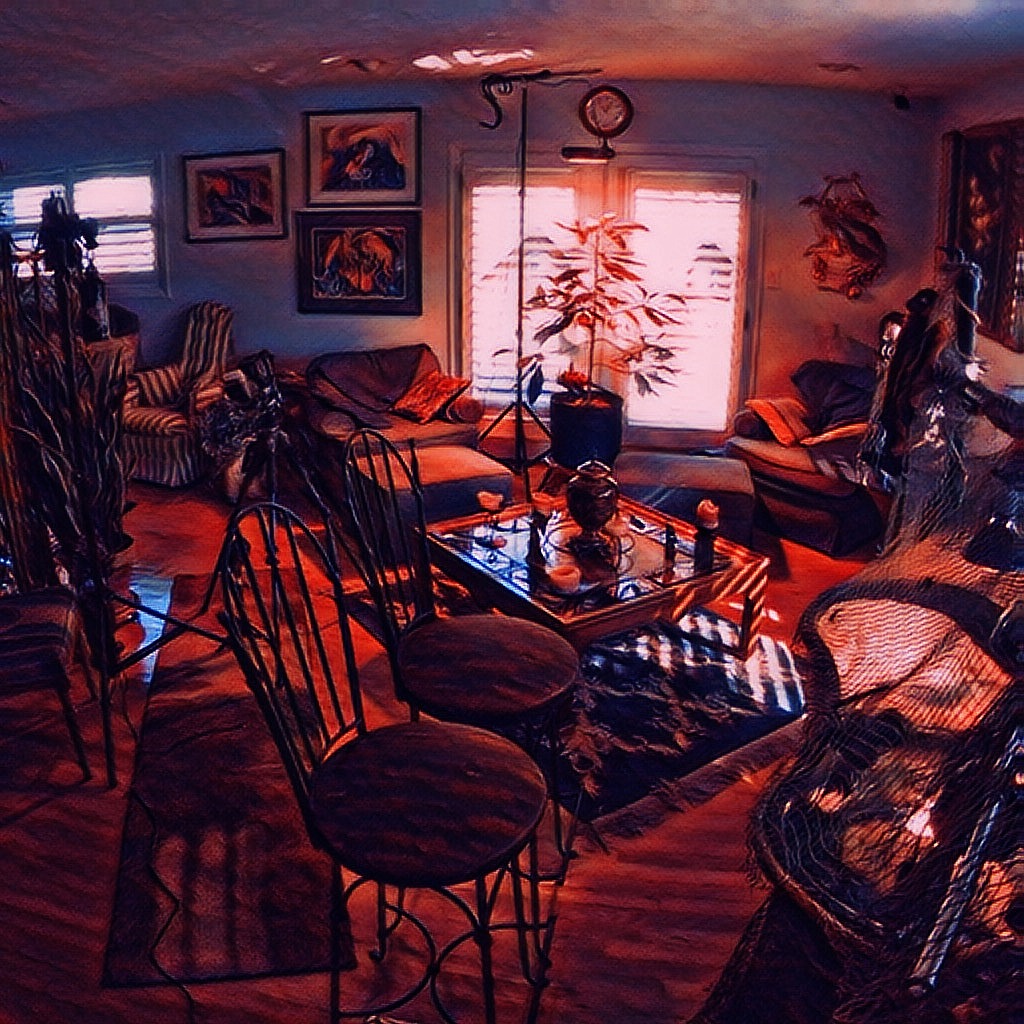This detailed painting portrays the interior of a stylish, intimate living room or restaurant, awash in artistic flair. The scene features a richly detailed hardwood floor, decorated with various carpets and rugs, creating a vibrant and textural base. In the center, a mirrored coffee table sits on top of one of these rugs, surrounded by multiple chairs, including wire ones, and plush sofa chairs near the windows.

The walls are adorned with framed and unframed artwork, giving the space an eclectic and cultured atmosphere. Several interesting pictures and a mask add to the unique decor, while a clock hangs above one of the windows. The room is bathed in natural sunlight from a window on the left and a sliding glass door towards the center, which, along with the light, creates a warm, inviting ambience with subtle red and pink tones.

Additionally, there's a plant situated in front of the window, further enhancing the cozy and lived-in feel of the space. The overall color scheme includes shades of brown, black, white, light blue, orange, and yellow, with most artworks and items appearing dark and muted. This captivating scene, likely to be admired in a household, captures the amalgamation of everyday comfort and artistic expression.